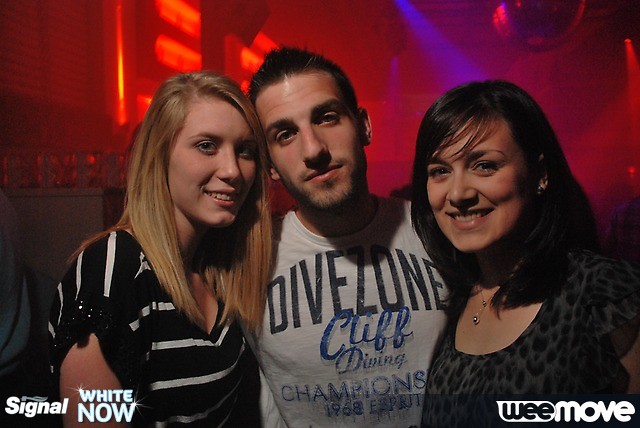In this nightclub scene illuminated by red and purple lights, a group of three friends stands together, smiling. On the left is a blonde woman with blue eyes wearing a black and white striped shirt. In the center is a man with short brown hair and some facial hair, donning a grey t-shirt that reads “Dive Zone Cliffs Diving Champions 1968.” To the right stands a brunette woman in a cheetah-print top, accessorized with a pearl necklace. A disco ball hangs from the ceiling amidst the vivid lighting, adding to the energetic atmosphere of the club. The image also features various logos and text overlays, with “Signal White Now” visible at the bottom left and “We Move” on the bottom right.